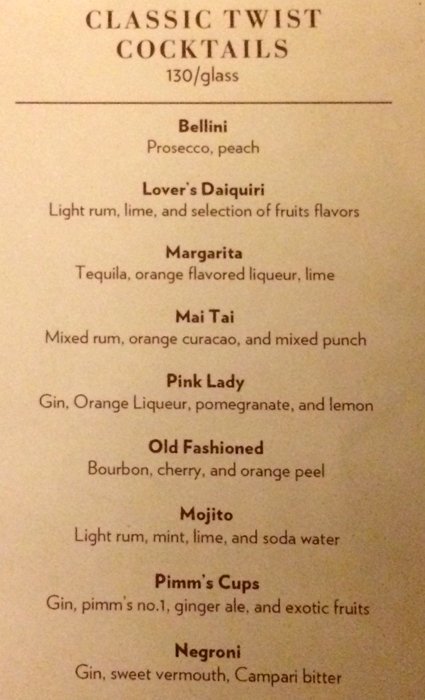The image depicts a tall, narrow cocktail menu in a portrait orientation, printed on a pale peach or off-white paper with a slight red or pink hue due to the lighting. At the top of the menu, "Classic Twist Cocktails" is printed in bold brown-black lettering, followed by the price "$1.30 a glass". The menu lists several cocktails from top to bottom, each in bold black ink with descriptions underneath in smaller letters. The cocktails include: 

1. **Bellini:** Prosecco and Peach
2. **Lover's Daiquiri:** Light Rum, Lime, and selection of fruit flavors
3. **Margarita:** Tequila, Orange Flavored Liqueur, and Lime
4. **Mai Tai:** Mixed Rum, Orange Curacao, and Mixed Punch
5. **Pink Lady:** Gin, Orange Liqueur, Pomegranate, and Lemon
6. **Old Fashioned:** Bourbon, Cherry, and Orange Peel
7. **Mojito:** Light Rum, Mint, Lime, and Soda Water
8. **Pimm's Cup:** Gin, Pimm's No. 1, Ginger Ale, and Exotic Fruits
9. **Negroni:** Gin, Sweet Vermouth, and Campari Bitter

The overall design is an illustration with typography, a graphic design style, and it is unclear if the menu is placed on a table or affixed to a wall.